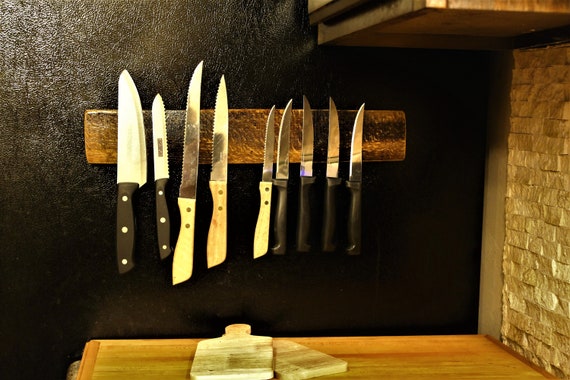The contemporary photograph features a kitchen scene dominated by a black wall, which houses a magnetic knife rack made from a bronze-colored rectangular piece of wood. The knife rack holds nine knives of various types and sizes, including butcher knives, serrated edges, steak knives, and paring knives. The handles of the knives vary from black plastic to light beige and wooden, all adorned with silver rivets. Below the knife rack, a mid-brown wooden counter with streaks of darker brown is visible, adorned with two light brown cutting boards with darker streaks, slanted against each other. To the right side of the image, a small backsplash of beige brick tiles is partially seen, alongside the base of a wooden cabinet cut off at the top. The photograph's dark setting, with its minimal natural light, emphasizes the contrast between the black wall, the bronze knife rack, and the lighter tones of the wooden counter and cutting boards.